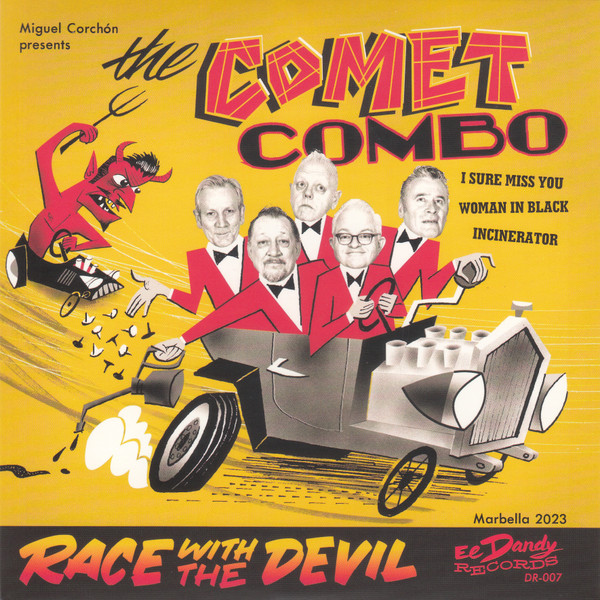The album cover for the vinyl record "Race with the Devil" by The Comet Combo features vibrant and eye-catching artwork that blends both cartoon and photographic elements. At the top of the square, dark yellow background, it reads "Miguel Corchon presents The Comet Combo" in bold, vintage-style red and black typography reminiscent of the 1960s.

The central image depicts a stylized, cartoony Tin Lizzy car in gray, with its motor exposed and the top removed. Inside the car are the band members, distinguished by their cartoon bodies dressed in red jackets, white shirts, and black bowties. Their faces, however, are black-and-white photographs, giving them a distinctive, hybrid look. The men appear to be in their 50s to 60s, adding a touch of authenticity.

Behind them, a menacing, cartoonish red devil with horns is in hot pursuit, driving a small black car and brandishing a pitchfork. The band members are not going down without a fight; one is dropping thumbtacks, and another is leaking oil to thwart their demonic pursuer.

To the right side of the image, song titles like "I Sure Miss You," "Woman in Black," and "Incinerator" are listed. Across the bottom of the cover, the album’s title "Race with the Devil" is prominently displayed in red and yellow letters. Below this, in smaller text, it states "Marbella 2023" and the record company information "E. Dandy Records DR-007.”